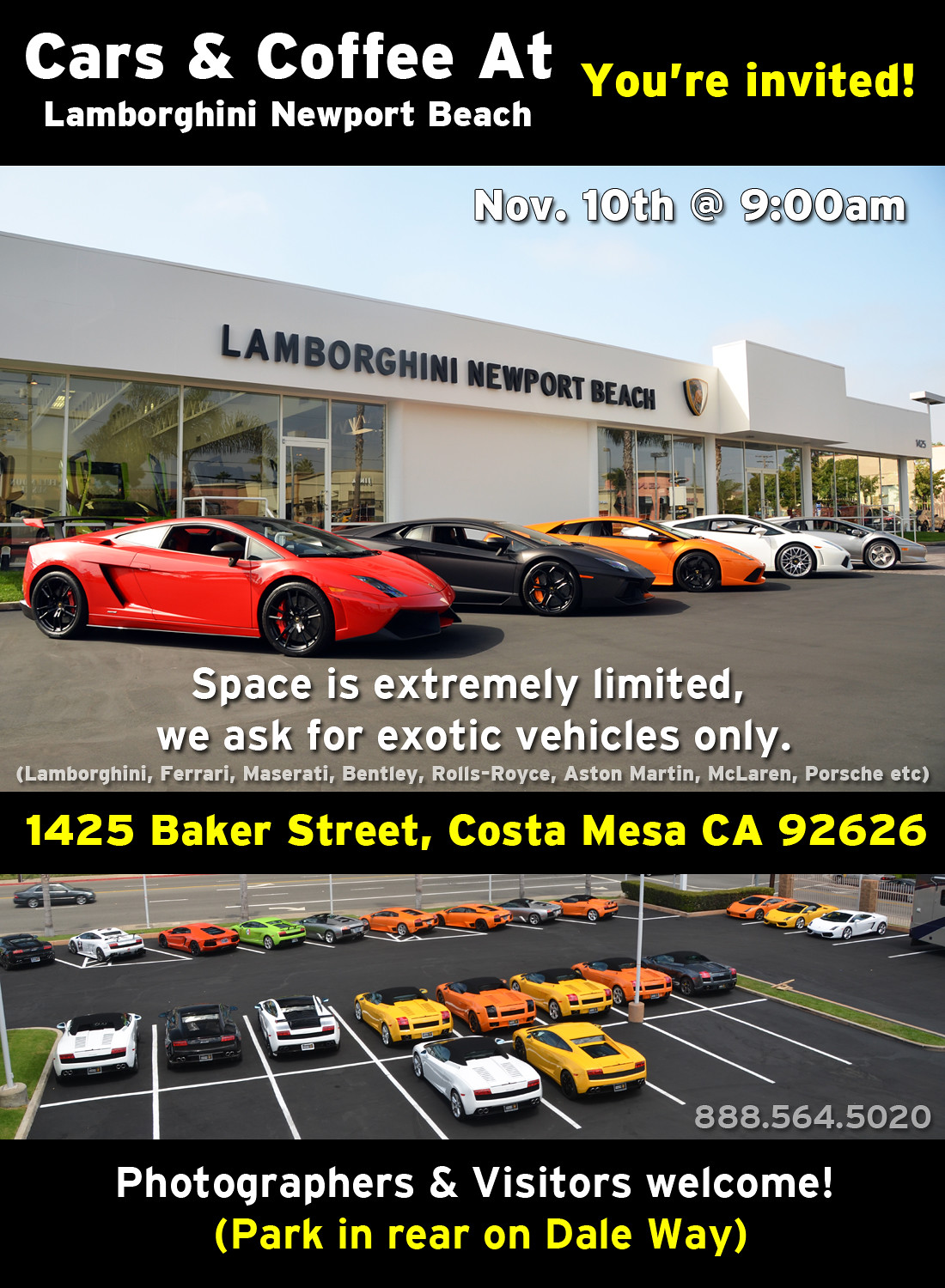The advertisement invites car enthusiasts to a "Cars and Coffee" event at Lamborghini Newport Beach on November 10th at 9 a.m., located at 1425 Baker Street, Costa Mesa, CA 92626. The top of the ad features a black background with white text, announcing the event, "Cars and Coffee at Lamborghini Newport Beach," with "You're invited" in yellow. Below, a photo showcases the front of the Lamborghini Newport Beach dealership with several Lamborghinis parked in front, including red, black, orange, white, and silver models. The text highlights that space is extremely limited, requesting attendees to bring exotic vehicles only (such as Lamborghini, Ferrari, Maserati, Bentley, Rolls-Royce, Aston Martin, McLaren, Porsche, etc.) in white text. Another photograph beneath displays a diverse collection of exotic cars in various colors parked on a blacktop surface. The ad concludes with a note in white text against a black background, stating, "Photographers and visitors welcome," with "Park in rear on Dale Way" in yellow.